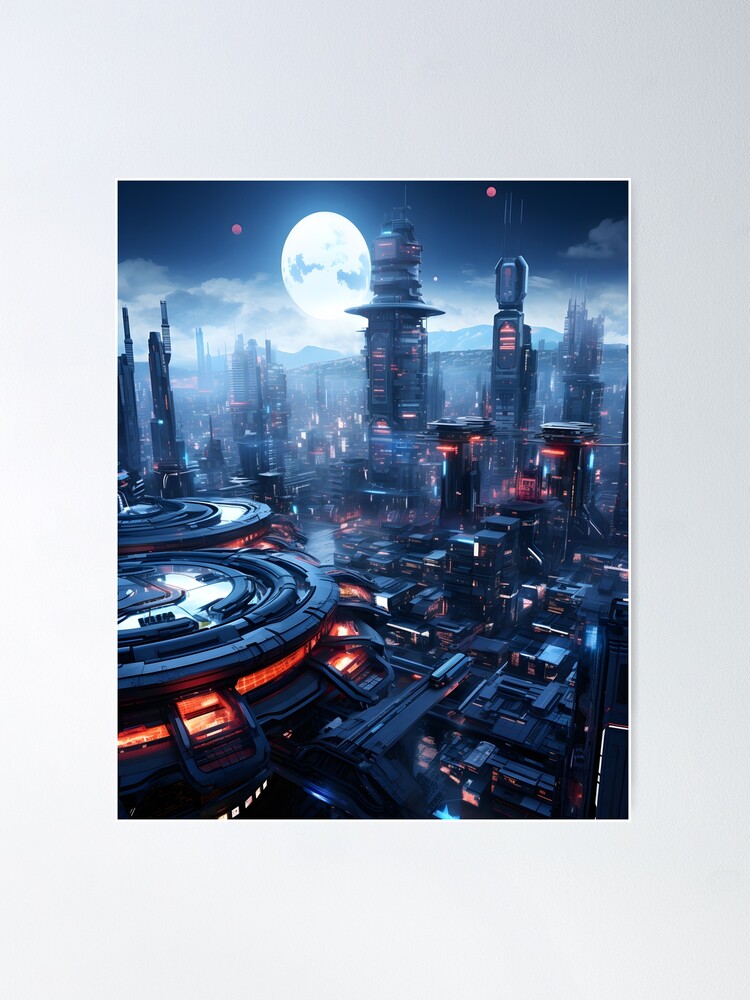This image presents a detailed sci-fi illustration of a futuristic cityscape, digitally created with vivid and striking colors. Dominating the scene is a large full moon, surrounded by a blue-hued, night-time sky interspersed with wispy white clouds. The city below is an intricate mix of towering skyscrapers, colored in shades of grey and blue, adorned with conspicuous red lights that resemble windows. These tall structures are complemented by shorter black buildings underneath and various grey buildings at the city's base.

On the left side of the image, two intriguing disc-like objects are visible, their tops reflecting a whitish-grey hue from what might be sunlight, and their sides are grey. Stairs appear to lead up to these objects, which also emit red lights. The bustling city includes moving vehicles, with some trains that are white and blue, adding to the dynamic futuristic ambiance.

In the distance, the city stretches towards the horizon, featuring hills and mountains beneath the vast, enormous moon - or possibly multiple moons. The immense celestial body bathes the entire cityscape in a luminous glow, enhancing the metallic and bright appearance of the structures. This elaborate depiction, set against an all-grey background, evokes a scene that feels several decades ahead or reminiscent of advanced Asian mega-cities, where architectural forms parallel the intricate designs of a circuit board.